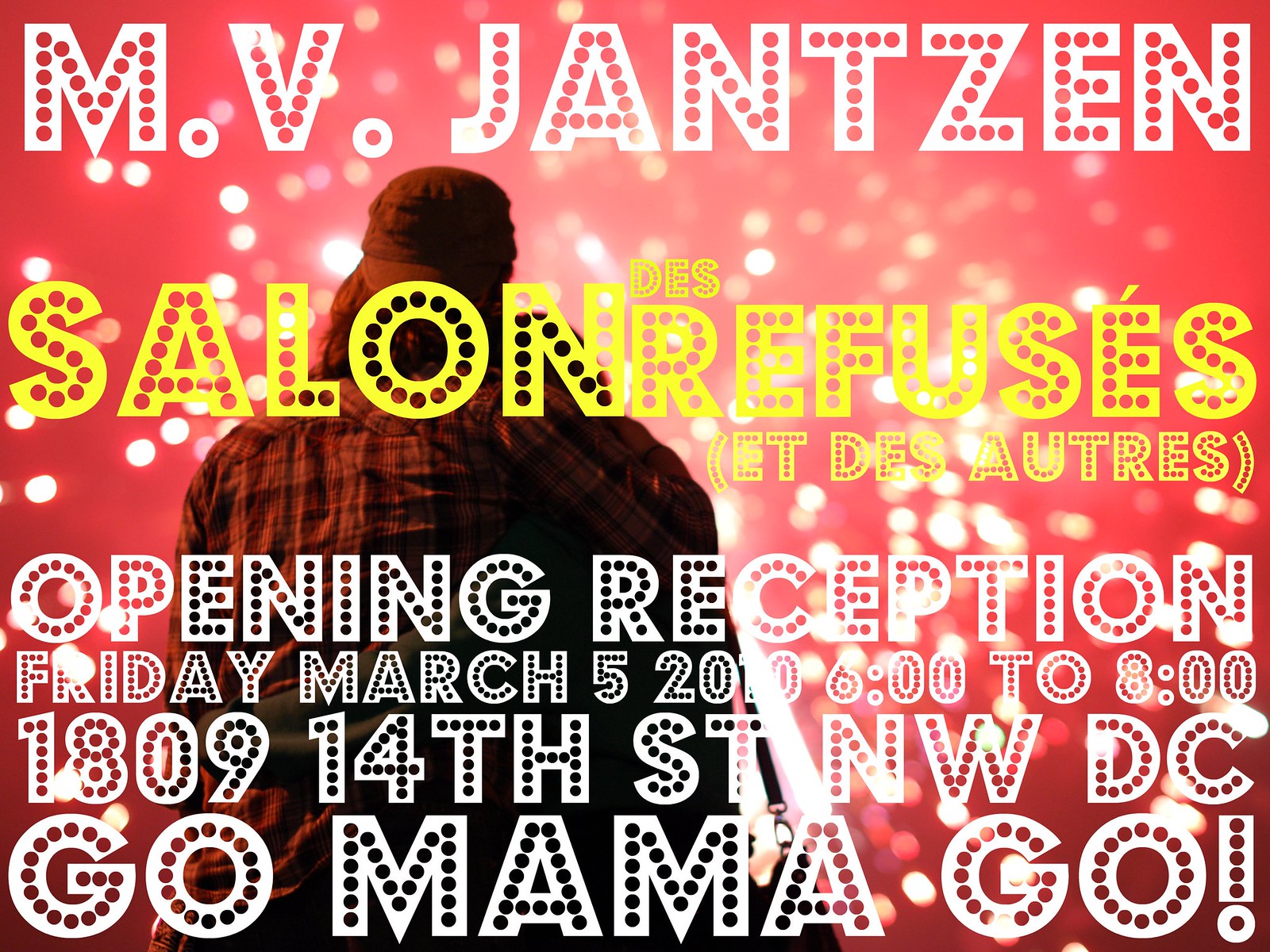The image is an advertisement for a studio or club event, with a vibrant and eye-catching design. The background is predominantly pinkish-red, decorated with white sparkles and circles, giving an impression of fireworks or twinkling lights. Central to the design is a photo of a large man standing slightly offset to the left, facing away from the camera. He is wearing a brown plaid shirt and a dark khaki backwards baseball cap, with long hair flowing down his back, seemingly looking into a crowd or performing on stage.

Superimposed over this dynamic background, bold and stylishly polka-dotted white text announces "MV Janssen." Beneath this, in contrasting yellow font, it reads "Salon Refuses." The details of the event are provided in white text with similar circle patterns: "Opening Reception Friday, March 5th, 2010, 6 to 8, 1809 14th Street Northwest DC." The flyer concludes with the enthusiastic phrase "Go Mama Go" at the bottom. This detailed, multi-layered design effectively conveys the excitement and energy of the upcoming event.